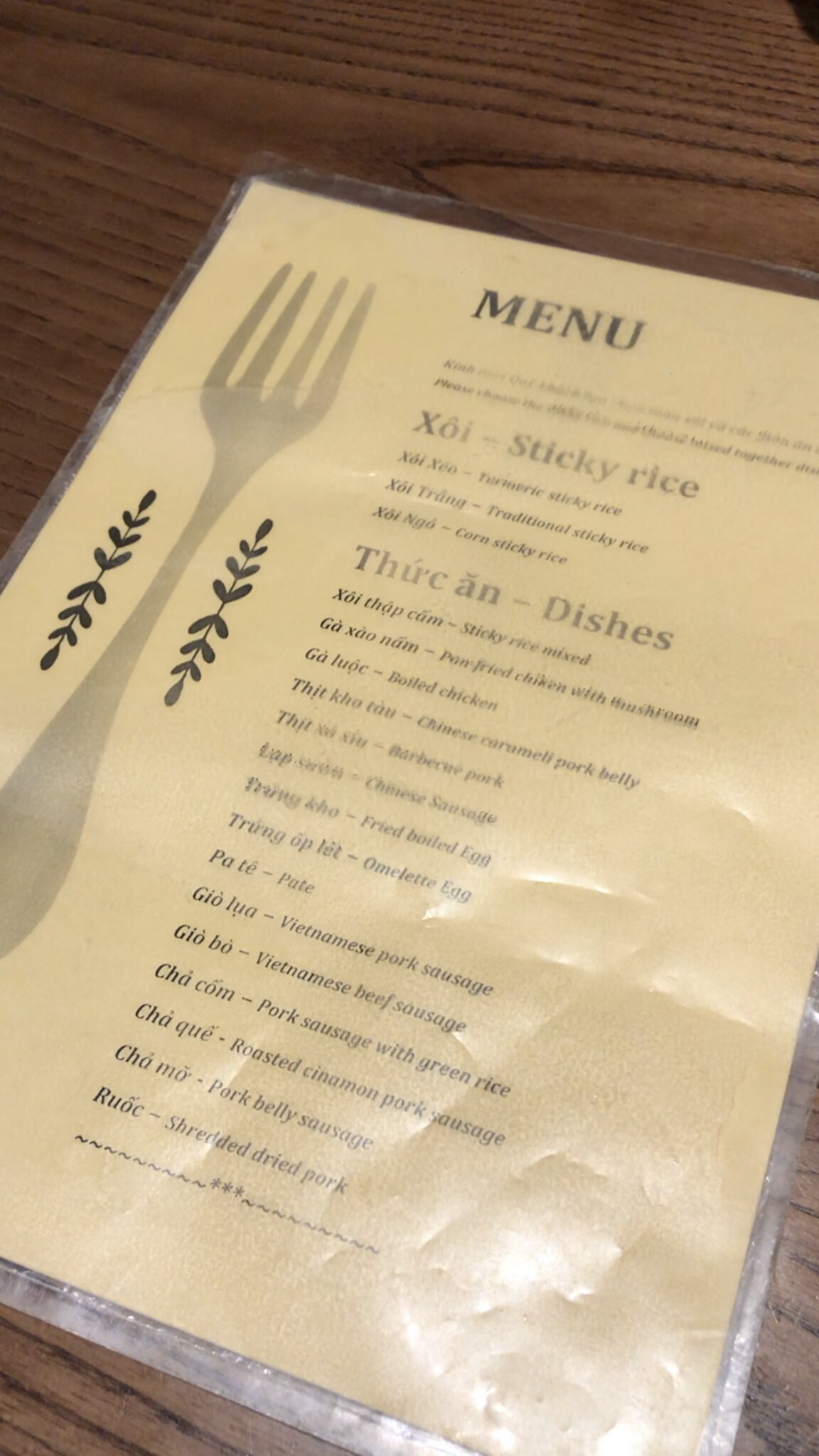This image captures the menu of what appears to be a Vietnamese restaurant, presented on off-white laminated paper. The left side of the menu is adorned with a simple illustration of a silver fork with four prongs, each handle featuring an elegant leaf pattern. The header prominently reads "Menu." 

The menu is divided into sections, starting with a section dedicated to sticky rice dishes, written in Vietnamese. This section lists three options. Another larger section lists 15 different dishes, also labeled in Vietnamese. The layout and design suggest an emphasis on simplicity and clarity.

The menu is placed on a wooden table with a visible wood grain pattern, adding a touch of warmth and rustic charm to the setting. The combination of the laminated menu and wooden table evokes a casual yet inviting dining atmosphere.